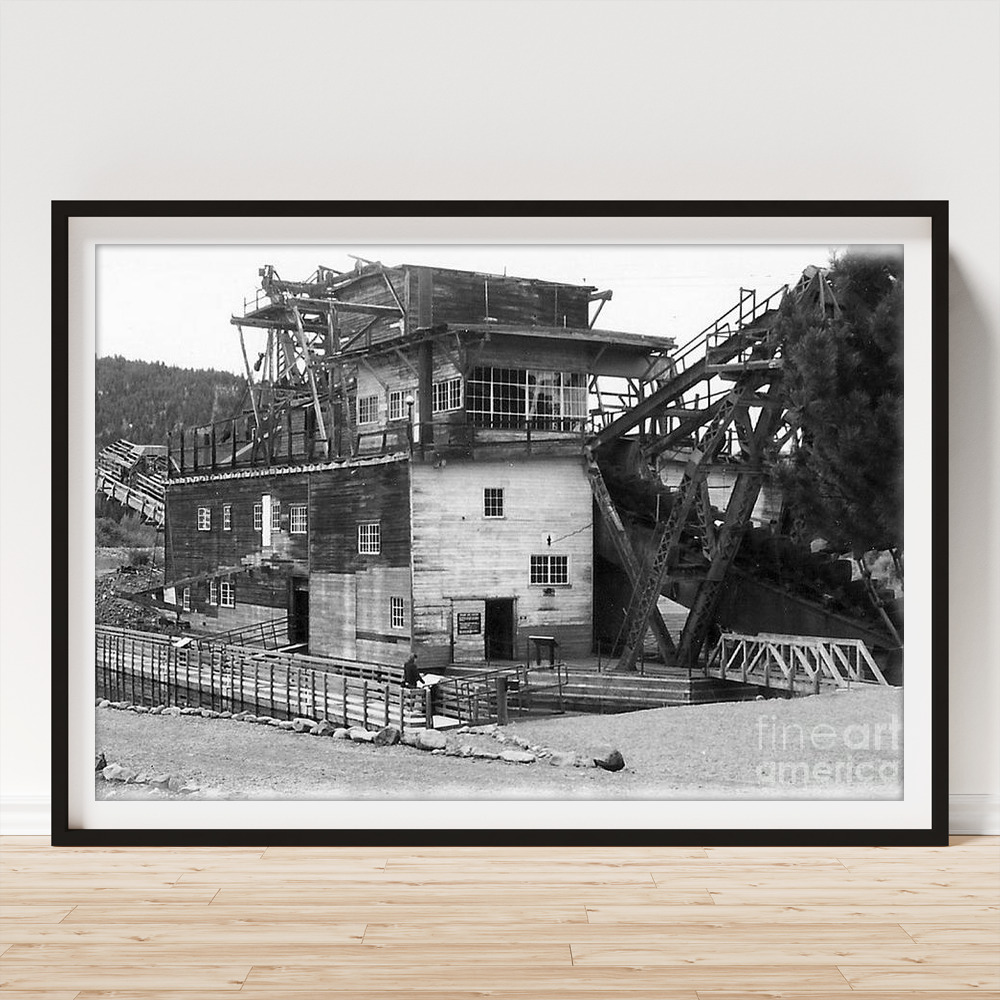The image depicts a black-and-white framed photograph resting against a white wall on a light-colored, bleached wood surface. The frame, likely black lacquer, shows a stark contrast with the bright setting. The photograph itself, occupying the top five-eighths of the overall canvas, is an antique scene marked as Fine Art America. The detailed and high-resolution image portrays an old, decrepit industrial building, possibly a mill or mining station, with three stories and numerous windows, some broken. Surrounding the structure is an assortment of debris, hinting at its dilapidated state. A pathway through dirt or possibly leading to water or a valley can be seen. Additionally, there are remnants of metal structures, such as beams or cranes, that are visibly falling apart. This historic building's observatory-like top floor, with several windows, punctuates its once industrious purpose.